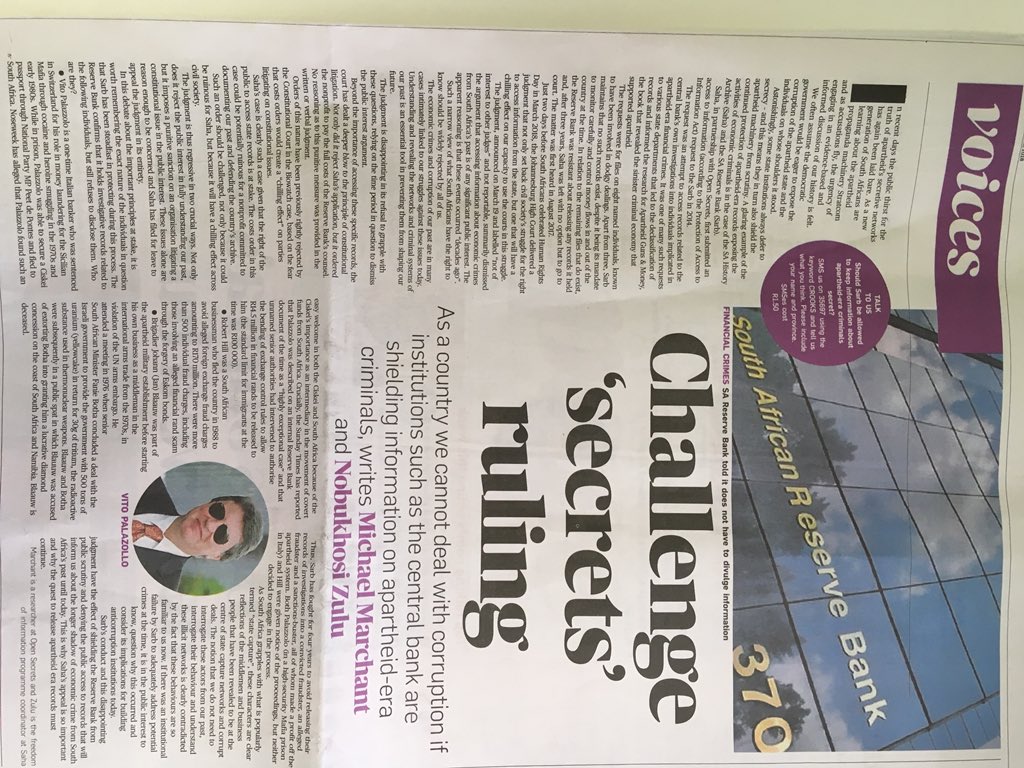The image depicts a page from a magazine or a news article, presented at an angle with the page turned sideways. The background is predominantly white. In the upper right corner, there is a purplish label with the word "Voices" written in white text. Directly beneath or adjacent to this label, "South African Reserve Bank" is inscribed in gold lettering. Additionally, the number "370" is also written in gold, possibly indicating a specific address or designation on an adjacent structure or context.

A prominent purple circle is noticeable, containing white text within it. Centrally located on the page, the large, bold text declares "Challenge Secrets Ruling." Below this headline, smaller black text provides more information, with certain names highlighted in purple for emphasis.

On the left side of the page, there is a photograph of a businessman. He is adorned in dark shades, a white shirt, a tie, and a black jacket. Surrounding him, there are various articles and texts, contributing to the overall dense composition of the page. Additionally, further articles and textual elements are present towards the top of the image, complimenting the extensive content of the page.